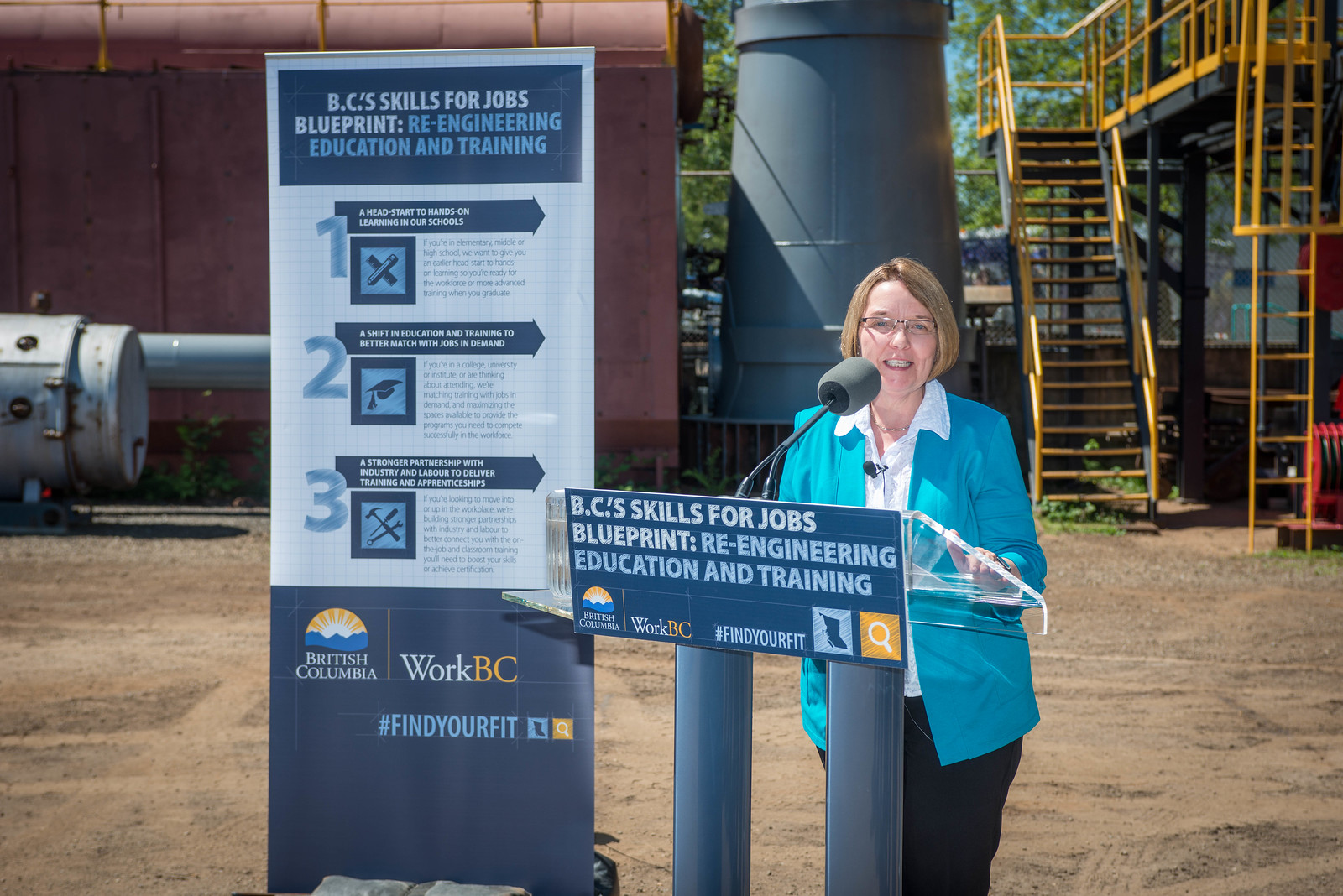In the image, there is an event taking place at what appears to be an industrial or agricultural facility, possibly an oil plant. A woman in her 40s is speaking behind a custom-made glass podium adorned with a banner that reads "BC Skills for Jobs Blueprint: Reengineering Education and Training." She is outfitted in a light blue jacket, a white button-up blouse, black pants, and glasses, with her hair styled in a coif cut above her shoulders.

The facility's background features various industrial elements, including a gray metal column or container, a metal containment box, a piece of machinery, and metal stairs leading up to a platform. There is also a yellow staircase and a yellow ladder visible on the far right.

Behind the speaker, additional signage provides further context: "Head Start to Hands-on Learning in our Schools," advocating for early hands-on education to better prepare students for the workforce and advanced training opportunities. The banners emphasize partnerships with industry and labor to deliver effective education and apprenticeship programs, aligning training with job market demands.

The event appears to be a dedication or announcement concerning an educational initiative in British Columbia, aimed at matching students with training and employment opportunities through practical, hands-on learning experiences.